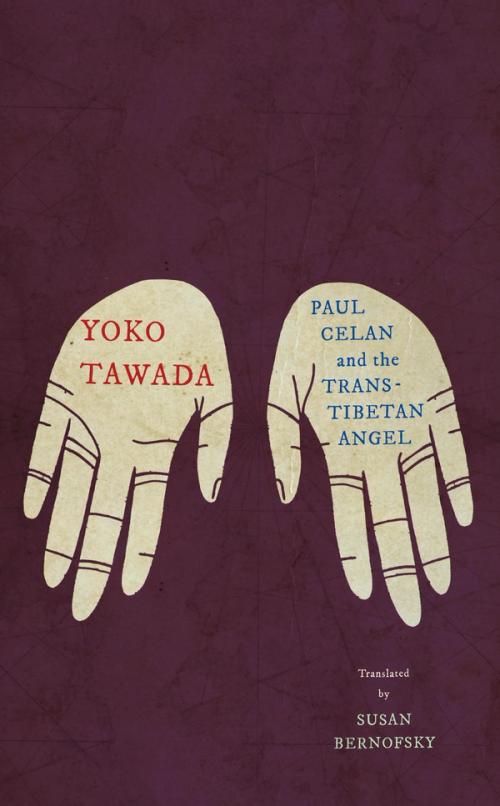The image is the cover of a book titled "Paul Celan and the Trans-Tibetan Angel" by Yoko Tawada, translated by Susan Bernofsky. The cover's background features a deep purple hue with a loose geometric pattern. Two pale yellow hands, pointing down with palms up and thumbs inward, are prominently displayed. In red, all-caps text, the author's name "Yoko Tawada" is written on the left hand. The right hand bears the book's title in blue text, with "Paul Celan" in all caps and "the Trans-Tibetan Angel" in uppercase on three lines. At the bottom right, "translated by Susan Bernofsky" is noted, with "translated by" in a white serif font and "Susan Bernofsky" in very light green or white text. The overall design is cartoon-like, adding a whimsical touch to the cover.